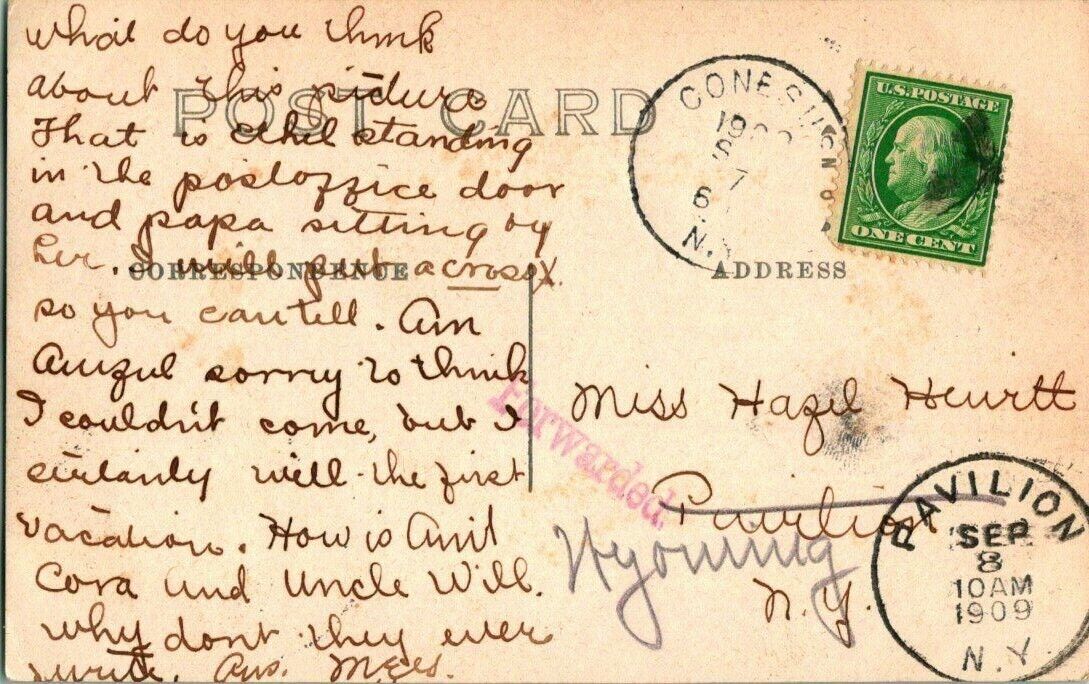This image is of the back side of a faded and yellowed postcard, dating from September 8th, 1909, as indicated by the stamp at the bottom right which reads "Pavilion, September 8th, 10 a.m., 1909, New York." Pre-printed at the top left are the words "Postcard," confirming its nature. A notable feature is the green U.S. one-cent postage stamp at the upper right corner, depicting Benjamin Franklin, which has aged gracefully. There are several ink stamps on the postcard, including one in faded pink that indicates it was forwarded at some point.

The left side of the postcard is adorned with a long and intricate handwritten message in cursive, likely penned in what was originally black ink that has since aged to brown. The detailed letter, albeit difficult to read due to the small cursive script, is addressed to "Miss Hazel Hewitt" and mentions details about family members and vacation plans. Among the text, one recognizable part reads: "What do you think about this picture that is something standing in the post office door and papa sitting by her? I will put a cross x so you can tell. Am something sorry? Think I couldn't come? How is something Cora and uncle will? Why don't they ever write something?"

Overall, the postcard, rich with historical value, serves as a snapshot of early 20th-century communication, adorned with period-authentic stamps and personal but now somewhat obscured reflections from over a century ago.